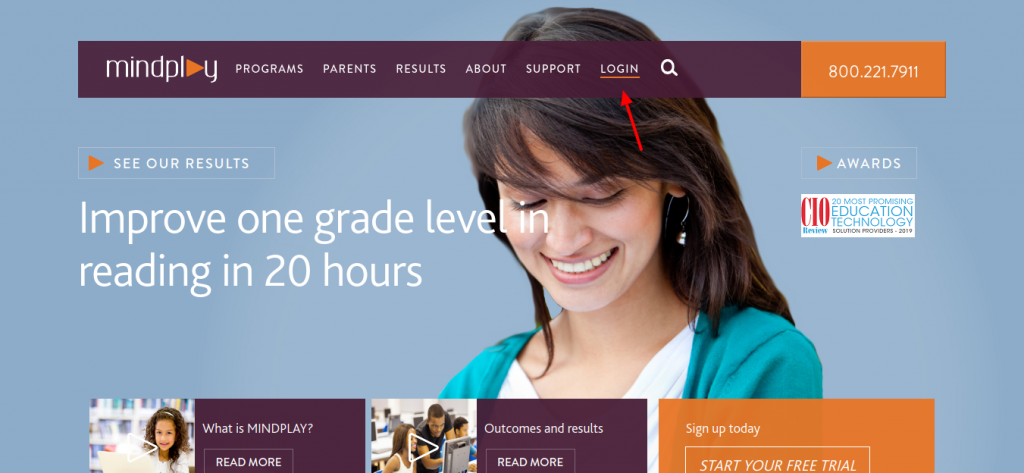Screenshot of the MindPlay website homepage. At the top left, the "MindPlay" logo is prominently displayed. To the right, there are navigation tabs labeled: Programs, Parents, Results, About, Support, and Login. A red arrow is pointing to the Login tab. On the far right, within an orange box, there is a contact phone number: 800-221-7911. Below the "MindPlay" logo on the left, the text "See Our Results" is visible, followed by the statement "Improve 1 Grade Level in Reading in 20 Hours." The background features an image of a smiling woman with brown hair and fringe bangs, looking down.